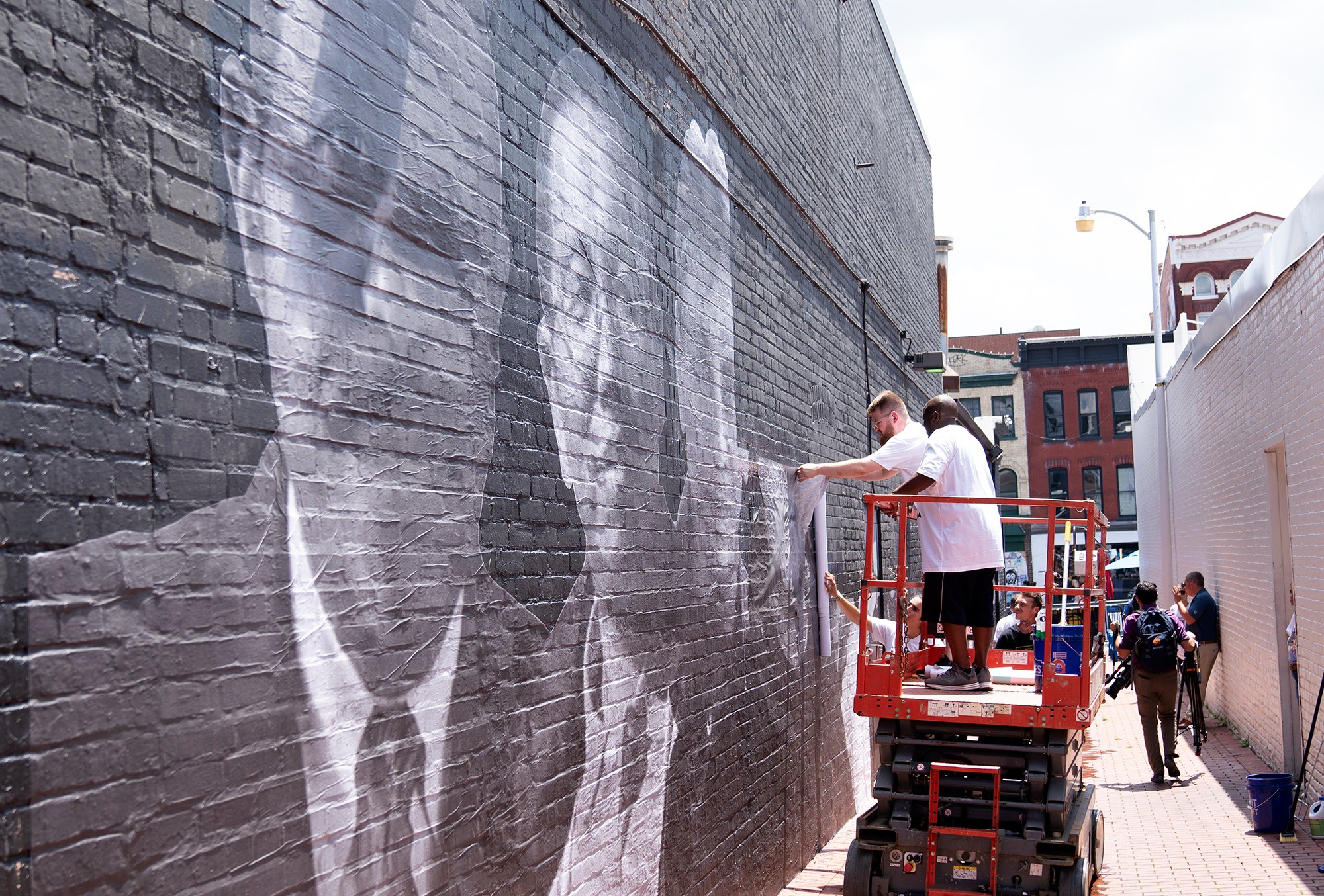The image captures a detailed scene of a mural in progress on the side of a brown brick building situated in an alleyway between two buildings. The mural depicts prominent men, potentially historical figures or civil rights leaders, dressed in suits and ties, reminiscent of a Mount Rushmore style. So far, two men's heads and shoulders are completed, and artists are actively working on the third figure. The artists, dressed in white shirts, stand on a small red hydraulic platform, which can be raised and lowered, visually marked by the visible black machinery part. The left side of the image shows an expanse of gray brick wall, narrowing diagonally toward the right. In the background, additional buildings and passersby are visible, emphasizing the mural’s urban setting. The close-up details hint that the mural may be created with pieces of wallpaper, as inferred from the material's appearance.